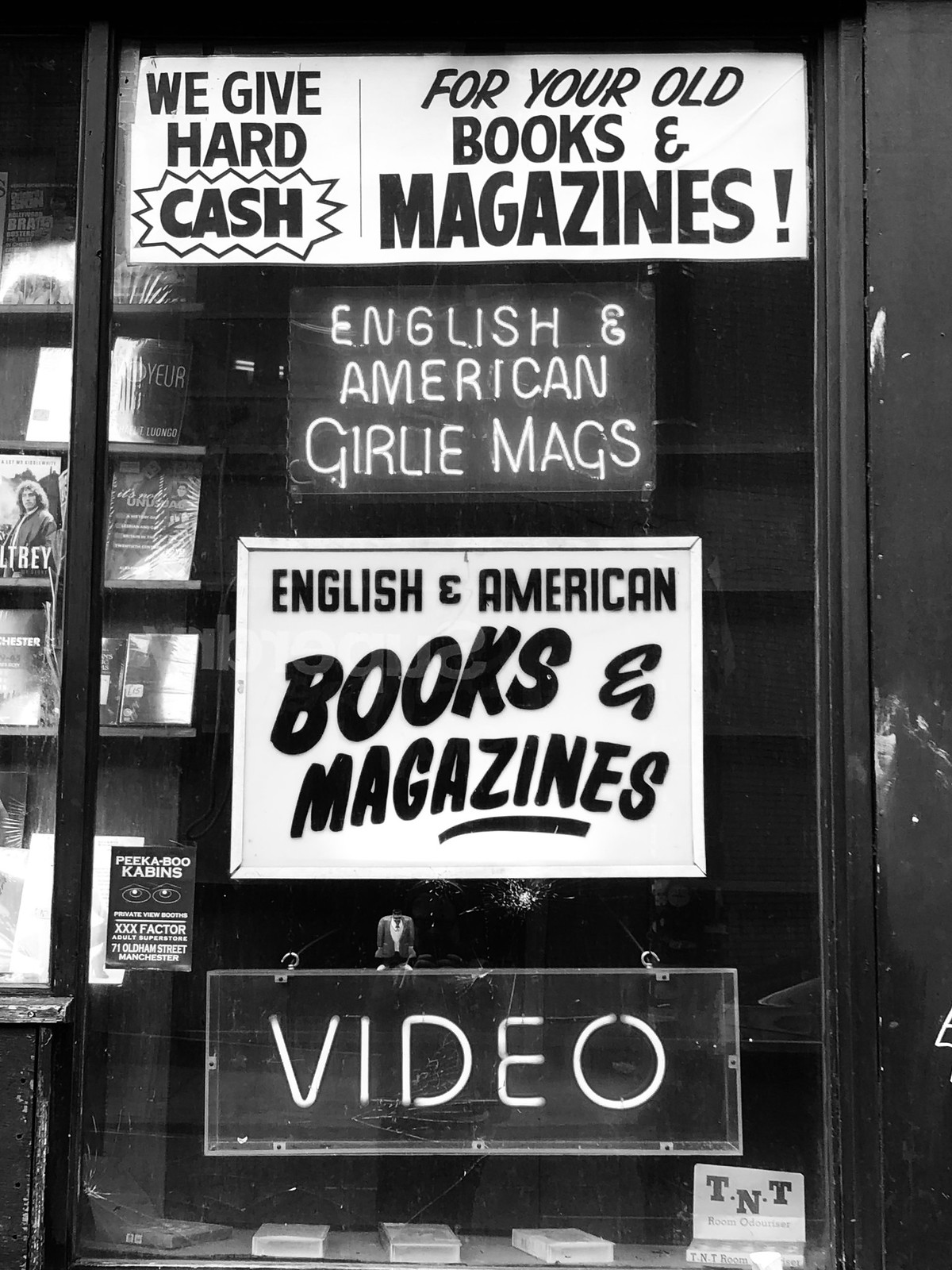This black-and-white vertical image captures a storefront window adorned with various signs. At the top, a white sign with black text declares, "We give hard cash for your old books and magazines!" Below this, a neon-style sign announces, "English and American girly mags." The next sign, also white with black text, states, "English and American books and magazines," underlined for emphasis. Further down, another neon sign, encased in glass, spells out "VIDEO" in uppercase letters. To the right of this sign is a smaller white sign with black lettering that reads "TNT." In the background, through the window, blurred titles of books like "Peekaboo Cabins" and "XX Factor" are faintly visible on the shelves, hinting at an eclectic collection inside. The overall aged appearance of the signs and the photograph itself suggests it might be an old or vintage bookstore.